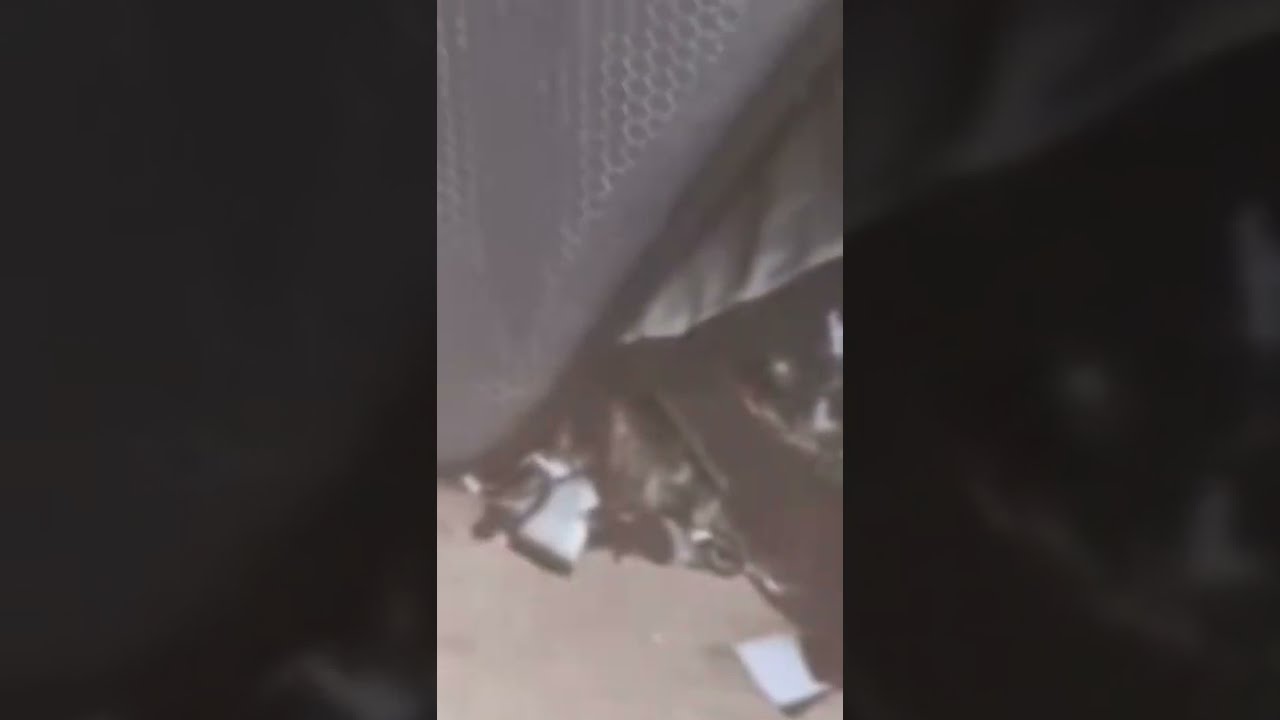The image consists of three panels: a central panel and two outer panels that are zoomed-in sections of the central image. The central panel is an underexposed and blurry black and white photo, difficult to clearly identify. It appears to show a pedal, possibly an accelerator, within a car complete with a metallic box beneath it, although it's obscured and cluttered.

The left and right panels are highly zoomed-in sections from the central image, focusing on the respective sides. Both panels are extremely dark and underexposed, adding to the difficulty in discerning specific details. Instead, they emphasize the chaotic and cluttered nature observed in the central image.

Upon closer inspection, the overall scene suggests an outdoor environment littered with trash and debris, including pieces of plastic, paper, and other miscellaneous garbage. The background features what looks like metallic grating or fencing in the upper portions of the panels, further hinting at an outdoor setting. The bottom of the image shows a beige, uncluttered surface resembling a floor.

In summary, the image depicts a blurry, underexposed triptych of what seems to be an outdoor area filled with trash and metallic structures, with a focus on a pedal-like object in a car at the center and intensified darkened sections on the sides.